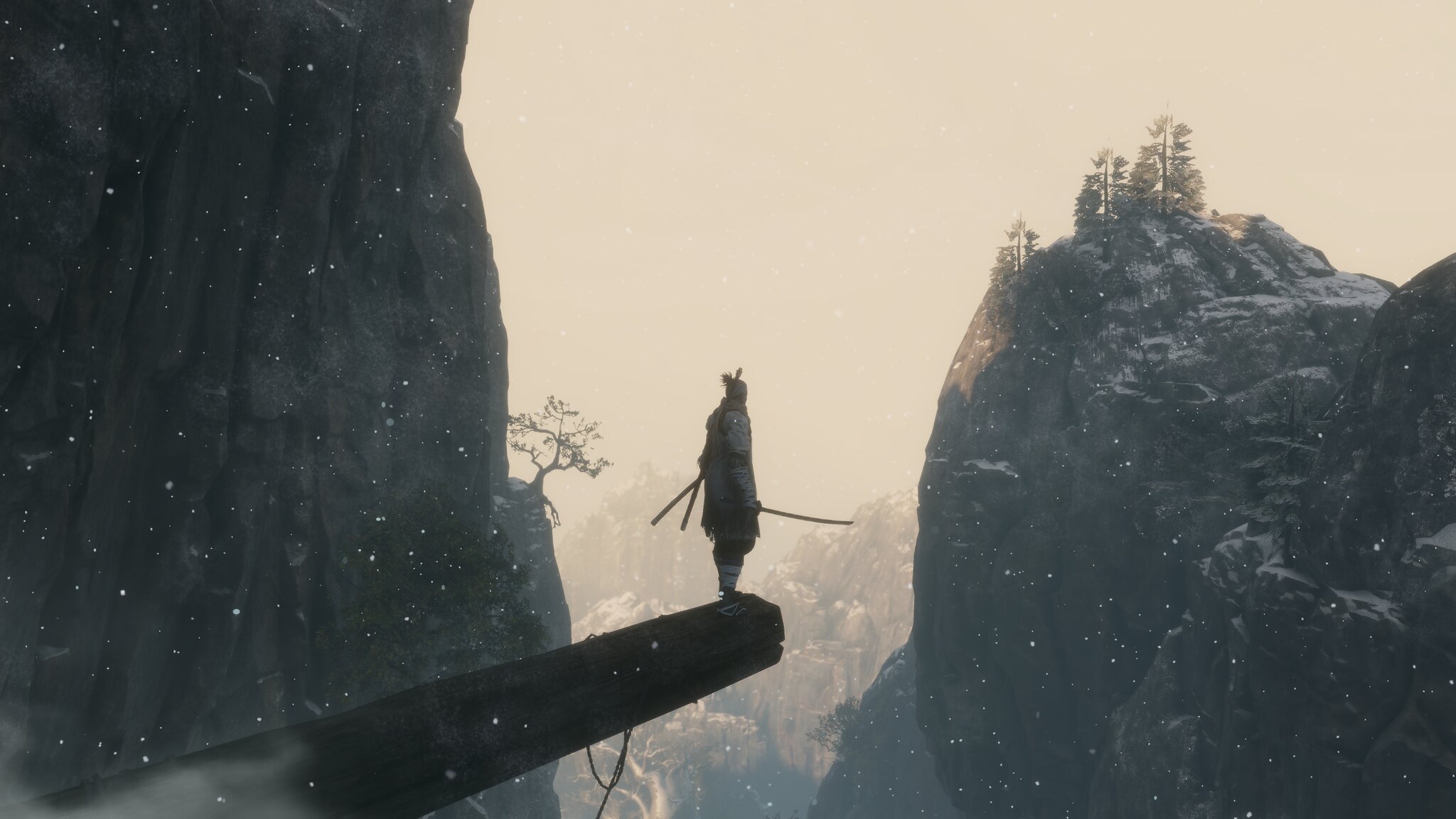This is a highly detailed computer-generated image depicting a dramatic mountainous landscape. Dominating the foreground is a rugged, wooden beam that extends precariously from the lower left corner of the scene out into a colossal abyss. Near the end of this beam, a solitary warrior, grasping a sword in their right hand, stands poised and contemplative. The character gazes out into the vast emptiness, where the ground drops away into an intimidating chasm that stretches hundreds or even thousands of feet below. To the left, on an adjacent cliff face, a solitary tree clings to the rocky terrain, its branches reaching out but remaining just beyond the warrior's grasp. In the broader view, the scene captures additional trees growing on a distant rock outcropping to the right, providing a stark contrast to the barren expanse between them. The image is wide-screen oriented, offering a panoramic glimpse of this epic, adventurous tableau.